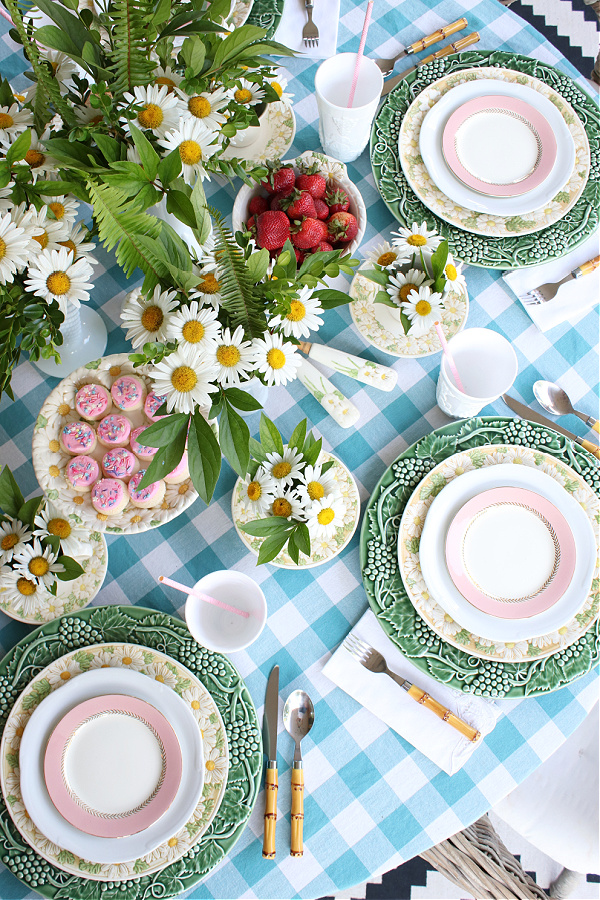The close-up, portrait-oriented image features a beautifully arranged dining table adorned with a blue and white checkered tablecloth. At each place setting, there is an elegant stack of plates: a large forest green plate with a textured edge reminiscent of grape vines, topped by a plate decorated with yellow daisies along the rim, then a scalloped edge white plate, and finally a smaller white plate with a pink border. Complementing the place settings, there are bamboo-handled forks, knives, and spoons, with napkins neatly placed underneath the forks.

In the middle of the table, several potted plants with white petal flowers and yellow centers add a touch of natural beauty. Additionally, the table is topped with white cups featuring pink straws, as well as a variety of colorful treats including pink-frosted cupcakes sprinkled with decorations, a bowl of fresh strawberries, and a plate of pink macarons.

The overall setting is vibrant, with the green, yellow, and white hues of the plates standing out among the colorful details around the table, creating an inviting and festive atmosphere.